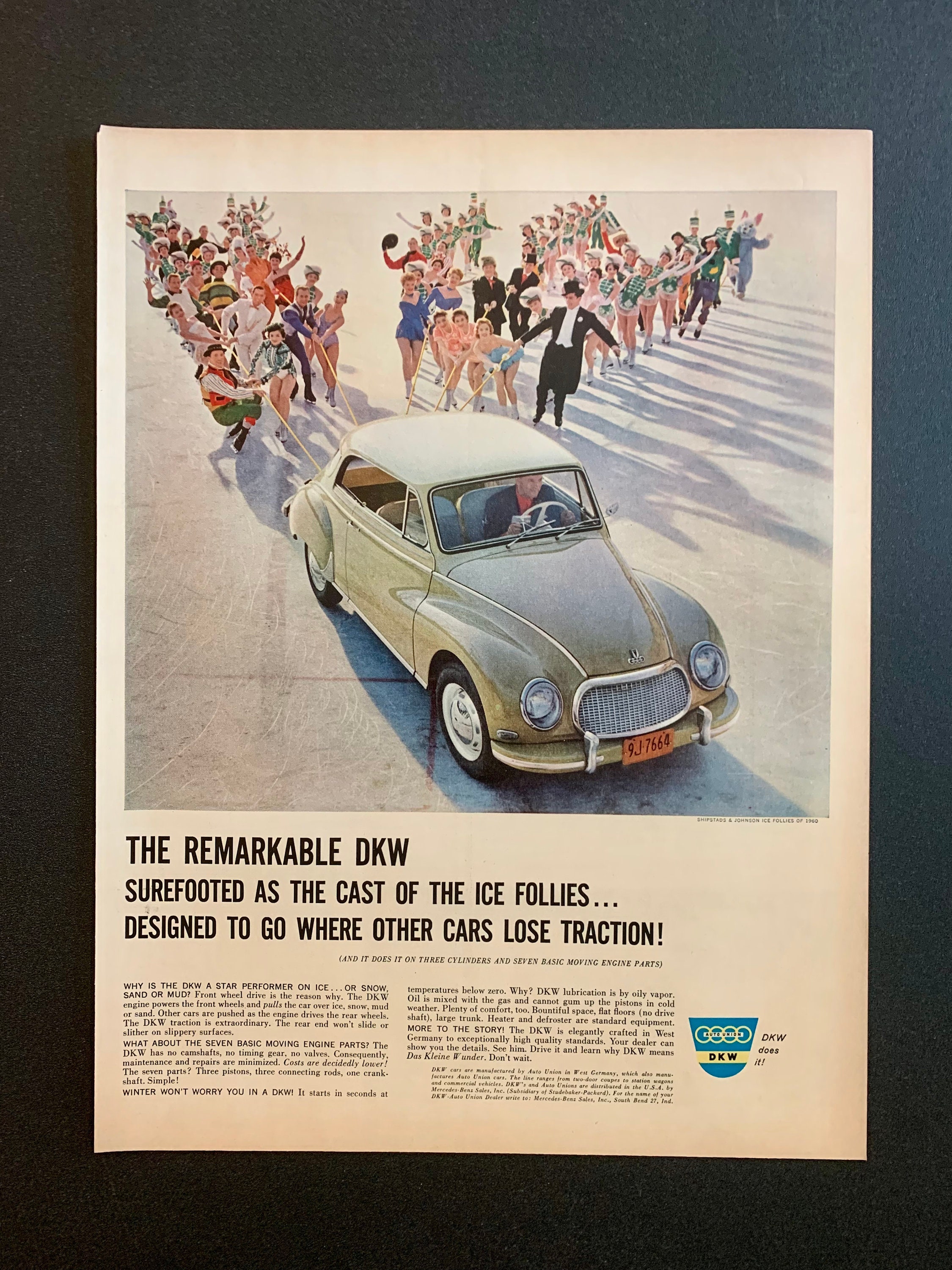The image, likely an advertisement from an older magazine possibly dating back to the 1940s or 1950s, features a distinctively olive green, two-door DKW car angled slightly to the right, facing the viewer. The car is driven by a man sporting a black blazer and a red shirt, gripping a large white steering wheel. Notably, the car has an orange license plate reading NJ7664. Behind the vehicle, there is a diverse array of people, including a music conductor, individuals in swimsuits, someone in a bunny costume, and band members, all pulling on ropes attached to the back of the car. The backdrop showcases these groups in various costumes emphasizing the car's reliability. The image is surrounded by a thick black border, with a prominent caption in the lower third: “The Remarkable DKW, sure-footed as the cast of the Ice Follies. Designed to go where other cars lose traction.” Additional text highlights its engineering prowess, stating, “...And it does it on three cylinders and seven basic moving engine parts.” A symbol in blue and yellow with the words, “DKW does it,” accompanies the detailed description.